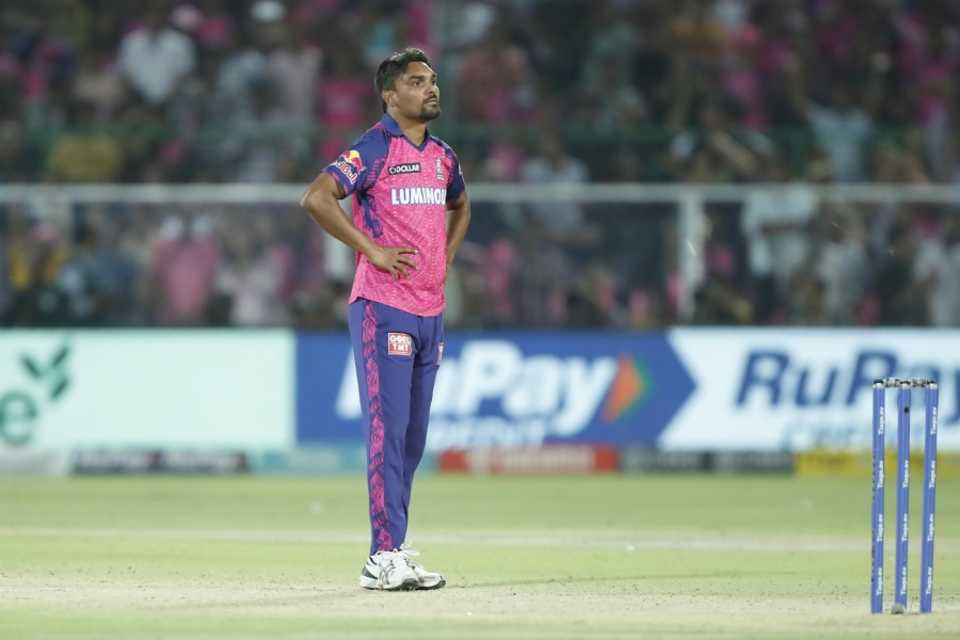In the image, a man stands confidently on a grassy cricket pitch with his hands on his hips. He has a dark complexion, black hair, and is dressed in a noticeable pink shirt with partially obscured text that appears to read "Luminol" and features blue short sleeves adorned with a logo on the right arm. His ensemble is completed with blue pants that sport a pink stripe down the sides and white athletic shoes. 

The cricket pitch is green and marked, although the exact details of the markings are unclear. At the edge of the pitch, a blue and white barrier displays the text "RU Pay" in alternating white and blue fonts, with a crowd of spectators blurred in the background. Near the man, a blue wicket stands with some white text, indicating the match setting. This outdoor photograph doesn't make it clear whether it was taken during the day or night.